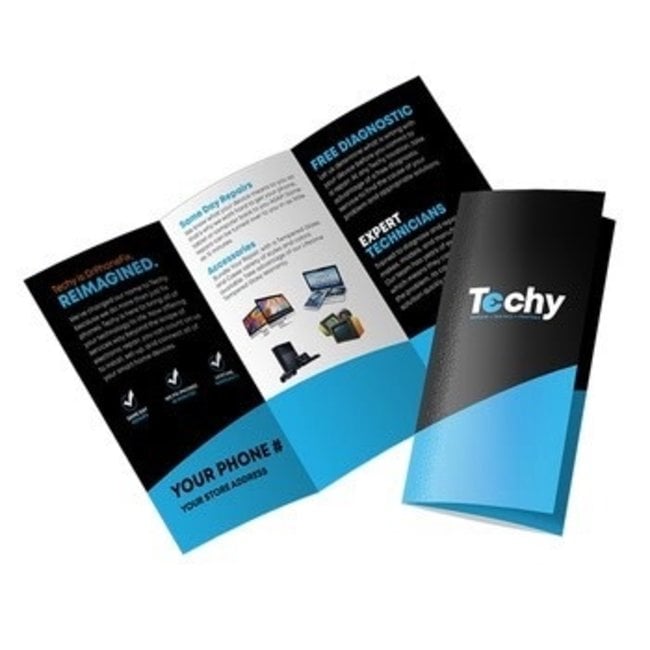The image features two Techie brochures set against a white background. The first brochure, which is closed and slightly folded, has a black and blue cover. The cover design includes a prominent white "T," a blue "E" that resembles a stylized "C" with a line through it, followed by "CHY" in white block letters. Below this, there is some unreadable blue text. The cover features a unique design with the top portion predominantly black, forming a near-rectangle with a small triangular extension, while the bottom section is blue in a triangular shape.

The second brochure is open, revealing three pages filled with blue and black text and imagery. The left page prominently displays the word "Reimagined" in dark blue, followed by some unreadable lines and three check marks. At the bottom of the open brochure, in black text on a blue background, it reads "your phone number" and "your store address." The middle page includes pictures of various technological devices such as a printer, laptop, desktop, and phone. On the far right panel, the brochure emphasizes "Free Diagnostic" on a black background with blue text and "Expert Technicians" in white on a blue background. Despite some unreadable segments, the brochure suggests it is promoting tech repair services, enticing customers with promises of free diagnostics and expert care.